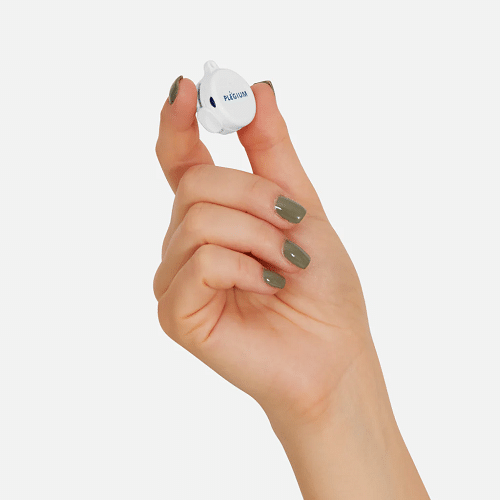The image features the right hand of a youthful female with manicured nails painted in an olive green shade. The hand belongs to a Caucasian person and emerges from the right side of a completely white background. She is holding a small, round white object between her thumb and index finger, with her other fingers naturally folded into her palm. The object, resembling a case like those used for ear pods, has a small latch and carries the word "plagium" written in light blue letters. The scene is minimalist, lacking any other elements or background distractions, possibly serving as an advertisement.